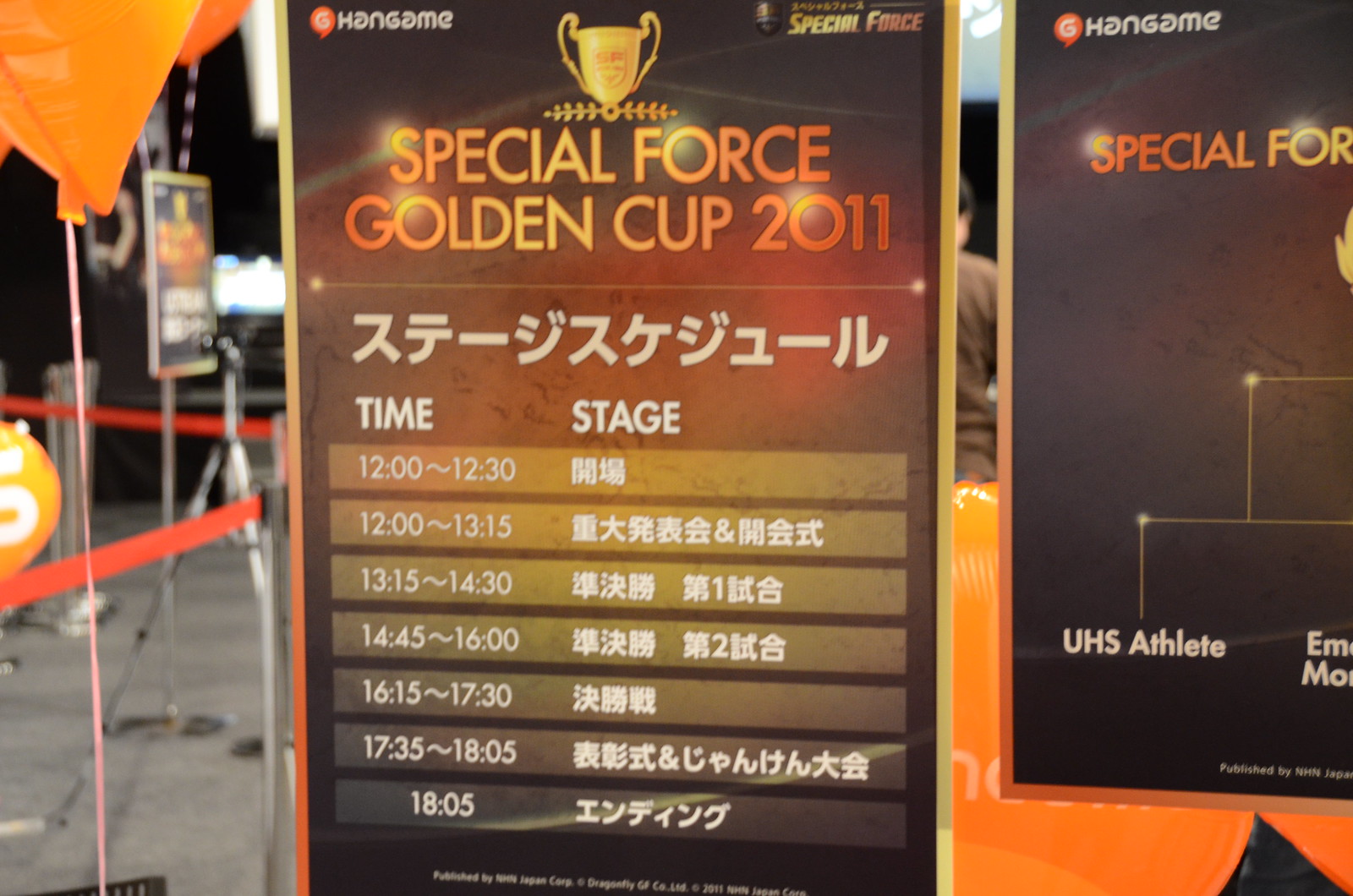In the center of the indoor photograph, there's a prominent sign featuring an artistic image of a trophy labeled "Special Force Golden Cup 2011." Below, the sign displays text in an Asian language, likely Japanese or Chinese, followed by a table divided into two columns. The first column is titled "Time" and lists various times in military format: 12:00 to 12:30, 12:30 to 13:15, 13:15 to 14:30, 14:45 to 16:00, 16:15 to 17:30, 17:35 to 18:05. The second column, labeled "Stage," consists of additional Asian characters. To the right of the main sign, there’s another partially visible sign that reads "UHS Athlete" alongside other text that is cut off and unclear.

In the background, a person can be seen standing amidst what appears to be a layout for directing foot traffic, marked with orange ribbons or velvet ropes. Additional signs and a few balloons are visible, possibly attached to the signage or the guiding ropes. The indoor floor seems to be a hard tile surface and there are various colors present in the scene, such as orange, black, brown, white, yellow, black, purple, pink, and blue. This setting is likely a convention or a similar organized indoor event.